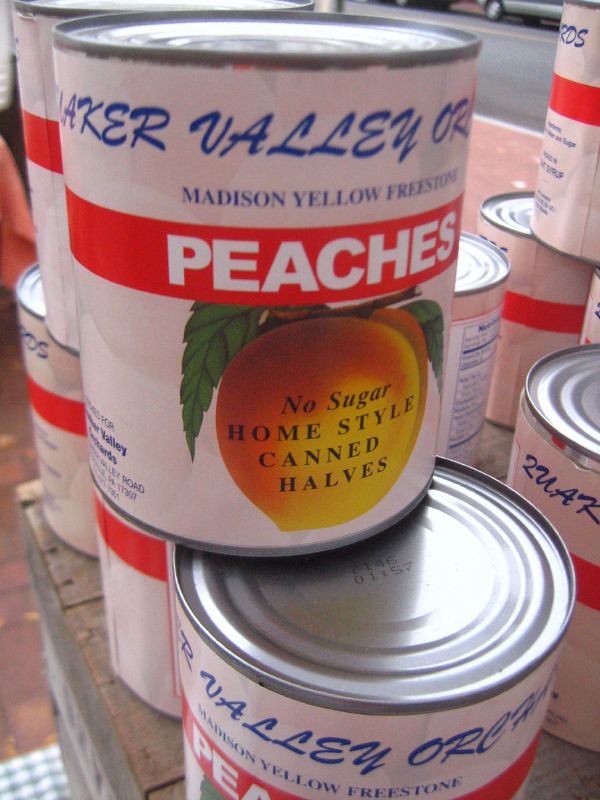The image showcases a scenic valley, possibly in New Jersey. Centered in the foreground is a stack of stone cairns, set against a dramatic precipice. The background reveals a coastline with sandy beaches and a view of the ocean. The scene includes a burst of colors with orange and green leaves decorating parts of the image. A figure wearing a yellow outfit stands out among blue stones and a prominent red rectangle adds a modern touch to the backdrop. Additionally, the word "beaches" is apparent on a white sign. At the bottom, a cluster of white and silver-lidded cans is stacked on a tiled floor, with reflections visible on their surfaces. A road meanders through the background, framed by white edges and various outdoor elements.